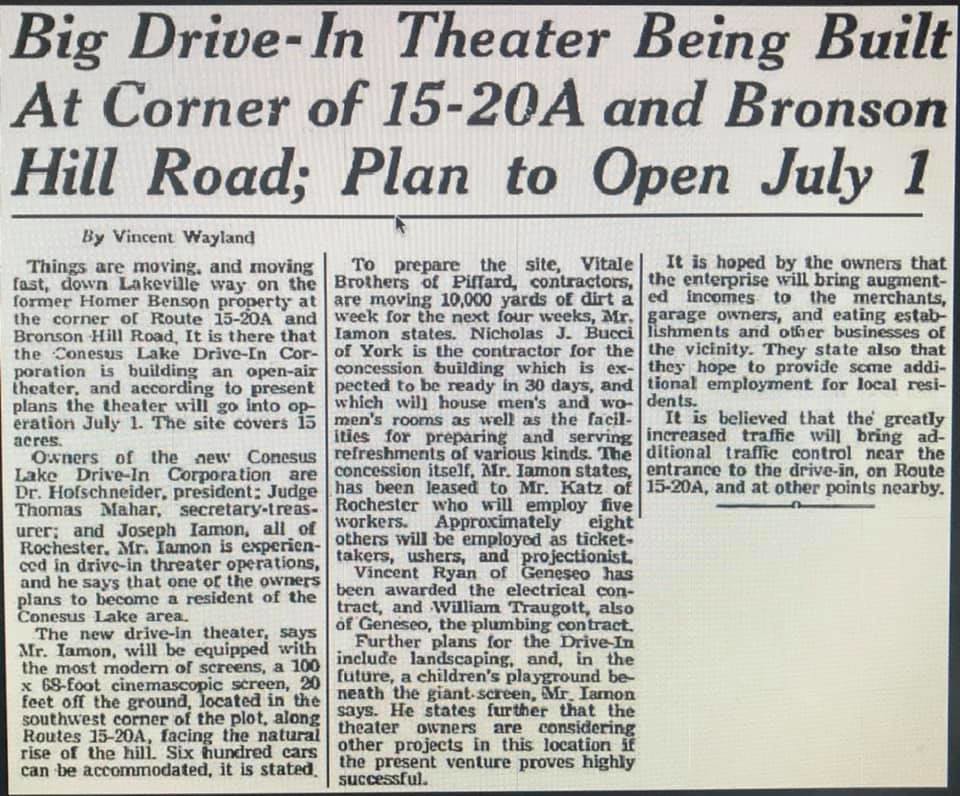This black-and-white newspaper article, printed on white background in landscape orientation, spans three columns. The bold headline stretching across the top reads: "A big drive-in theater being built at the corner of 15-20A and Bronson Hill Road. Planned to open July 1st. By Vincent Whalen." The article describes rapid developments on the former Homer Benson property at Route 15-20A and Bronson Hill Road, where the Kinesis Lake Drive-In Corporation is constructing an open-air theater set to open on July 1st. The site, covering 15 acres, is a bustling project that's moving fast. The vintage style of the article and the presence of an online mouse marker add to its historical and digital context.